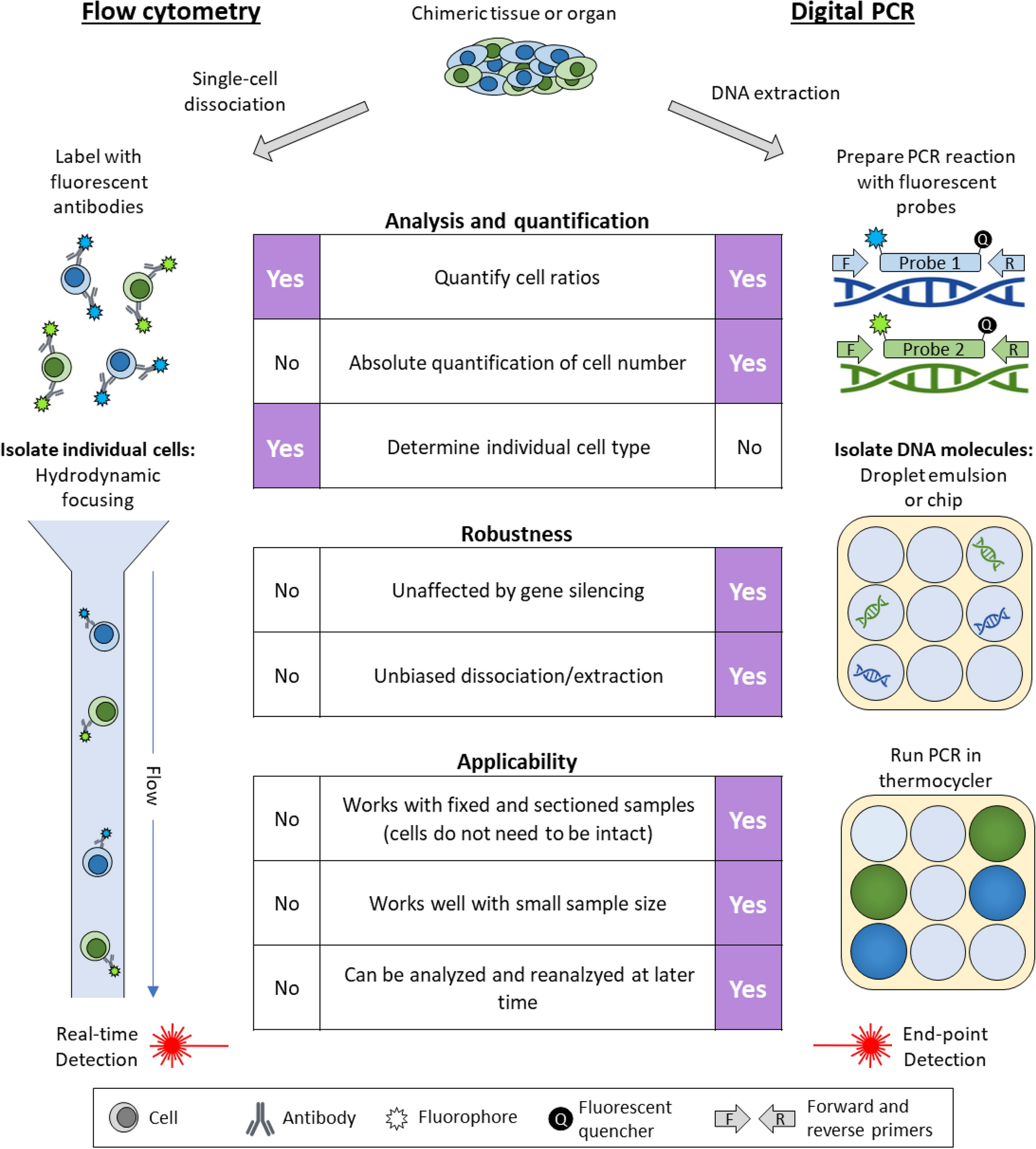The image depicts a detailed flowchart contrasting two scientific methods: flow cytometry on the left and digital PCR on the right, both aimed at analyzing chimeric tissues or organs. At the top, the chart starts with "Chimeric tissue or organ," which then branches into two distinct processes.

For flow cytometry, the process begins with single cell dissociation, followed by labeling the cells with fluorescent antibodies, which are illustrated with small circles attached to the cells. The next steps involve isolating individual cells through hydrodynamic focusing, depicted with a blue beaker and tube containing cells. This is followed by real-time detection using a laser. 

For digital PCR, the process starts with DNA extraction. It then involves preparing the PCR reaction with fluorescent probes. Subsequent steps include isolating DNA molecules using droplet emulsion or a chip, running PCR in a thermocycler, and endpoint detection.

Between the two methods, there are three sections labeled Analysis and Quantification, Robustness, and Applicability. Each section evaluates various criteria for both methods with "yes" or "no" answers:
- Analysis and Quantification: quantified cell ratios ("yes" for both), absolute quantification of cell numbers ("yes" for digital PCR, "no" for flow cytometry), and determination of individual cell types ("yes" for flow cytometry, "no" for digital PCR).
- Robustness: unaffected by gene silencing ("yes" for digital PCR, "no" for flow cytometry).
- Applicability: unbiased dissociation/extraction ("yes" for digital PCR, "no" for flow cytometry), works with fixed or sectioned samples where cells do not need to be intact ("yes" for digital PCR, "no" for flow cytometry), works well with a small sample size ("yes" for digital PCR, "no" for flow cytometry), and can be analyzed and reanalyzed at a later time ("yes" for digital PCR, "no" for flow cytometry).

At the bottom of the chart, there's a legend indicating symbols used to represent different elements such as cells, antibodies, fluorophores, fluorescent quenchers, and forward/reverse primers.